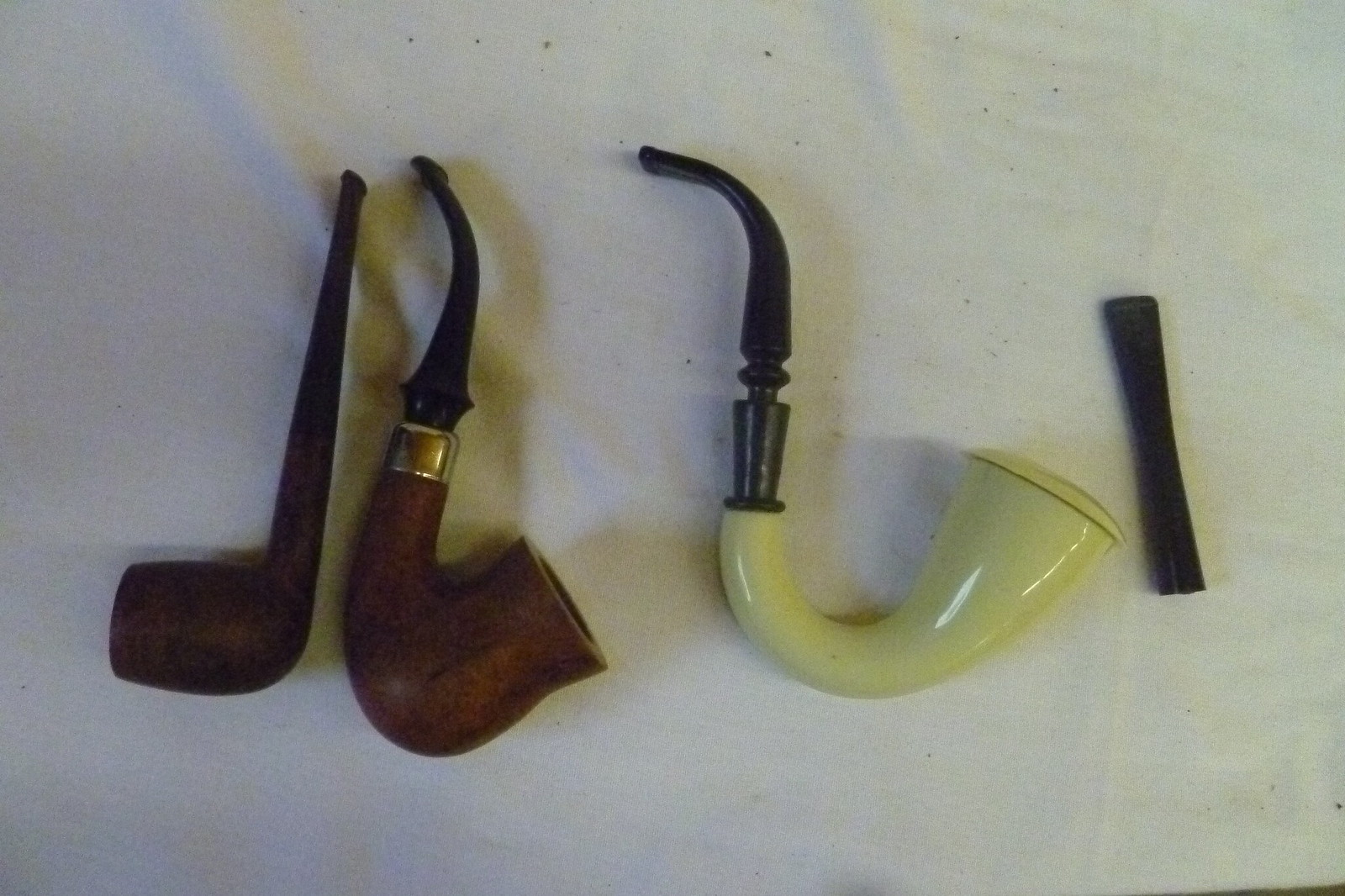This detailed photograph showcases a collection of vintage smoking pipes laid out on a slightly wrinkled, white tablecloth, which has a few specks of debris or crumbs scattered across its surface. The photo features four objects, all appearing to be antique smoking pipes, each with unique characteristics. 

On the far left, there is a simple, straight pipe made of wood with a horizontal tube where smoke would escape. This pipe is primarily brown. To the right, the second pipe is more intricate with a curved body; it has a dark brown wooden color with a gold band in the middle and a black section at the mouthpiece. The third pipe is distinct with a longer, more pronounced curve. It starts with a black handle and transitions into a cream or ivory-colored body, featuring a black mouthpiece. 

The final object on the extreme right is a small black cylinder, which appears to be a detached mouthpiece, lying separately from the rest. Each pipe's unique design and color contribute to the vintage and antique aesthetic of the collection captured in this image.